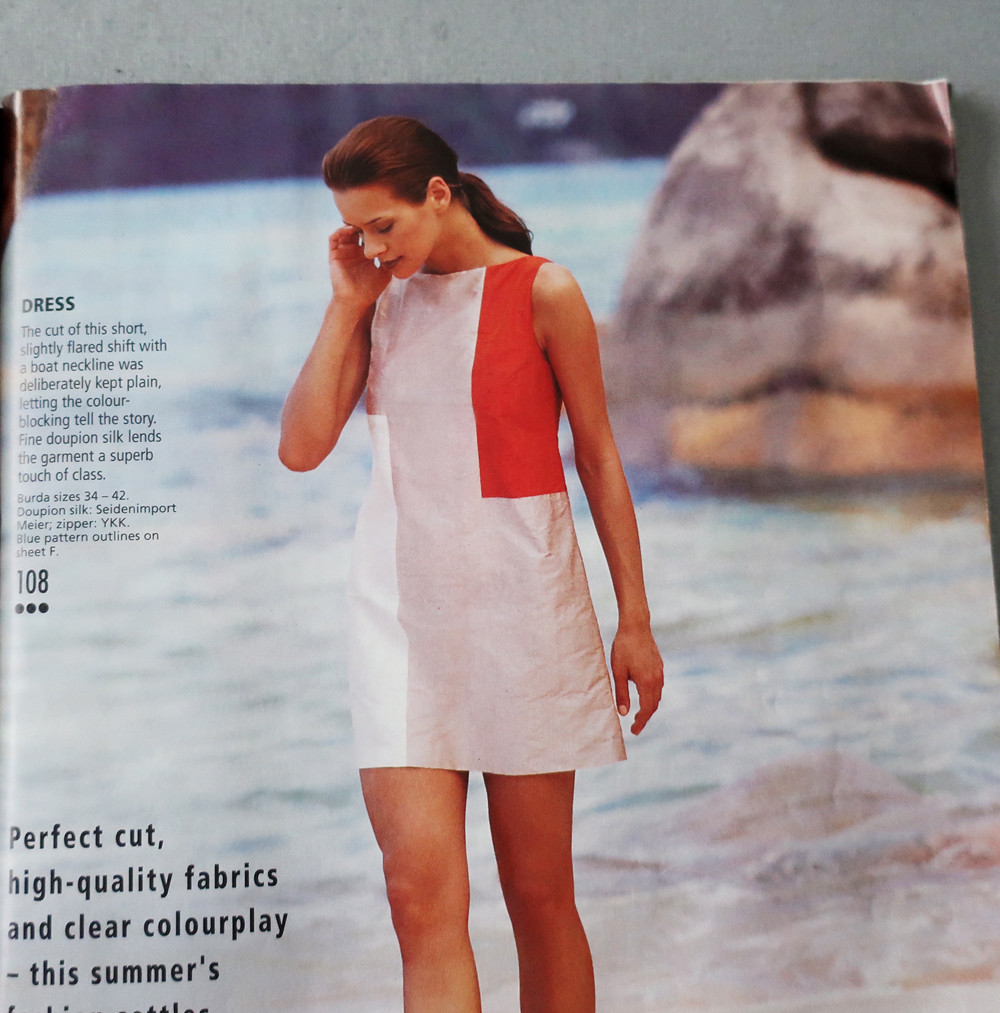The image is a square photograph of a corner of a fashion magazine, positioned in the top right of the frame. The magazine showcases a model standing on a beach shore, with a light blue body of water and a large, smooth gray rock in the background. The model is tall, has light skin, and dark brown hair tied into a ponytail. She is wearing a color-blocked dress that features segments of white, light pink, and red. The dress is visible from her calves up, and she is facing forward with her head tilted downward to the bottom left corner. The scene includes soft reflections in the water, giving it a serene, blurred backdrop. Printed on the left side of the magazine page, in fine text, are details about the dress, including sizes and style information. At the bottom in larger black letters, the text reads, "Perfect cut, high-quality fabrics, and clear color play, this summer's," though the sentence is cut off at the end. The magazine is laid on a gray table.